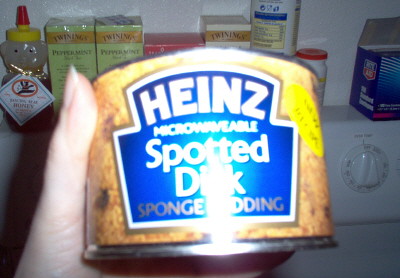In the image, a hand with visible white skin and a discernible fingernail is holding a Heinz brand microwavable sponge pudding. The sponge pudding, still in its original packaging, features a blue logo typical of Heinz, although glare obscures part of the logo and a mysterious sticker whose text is illegible. The pudding itself appears tan-ish brown with dark spots. In the background, there is a shelf filled with various boxes or jars stacked alongside each other. These items rest on what appears to be a cooking surface, complete with an indistinct knob that might belong to a stove.